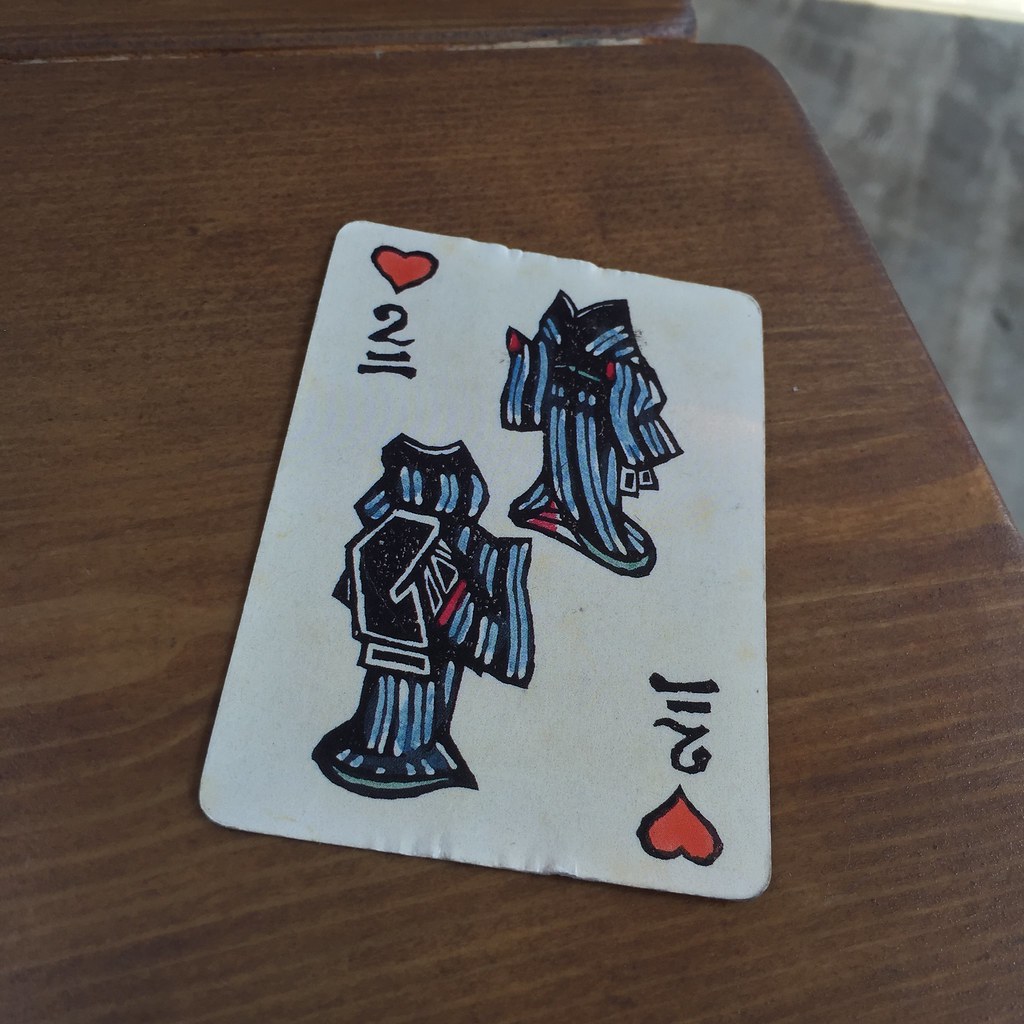This is a color photograph of a homemade or DIY playing card, designed to mimic the size and shape of a standard playing card. The card appears to be constructed from thin white paper, evidenced by its slightly crinkled top and bottom edges. At the top and bottom margins, a red heart outlined in black is prominently featured. Below each heart, the numeral "2" is drawn with double underlines beneath it. The center of the card showcases an illustration of an empty flowing gown, reminiscent of traditional Chinese or Japanese attire. The gown is adorned with blue and black stripes, along with subtle red detailing, although no figure is depicted wearing it. The overall aesthetic suggests a careful but amateur artistic effort, capturing the essence of a traditional playing card with a unique, personal touch.